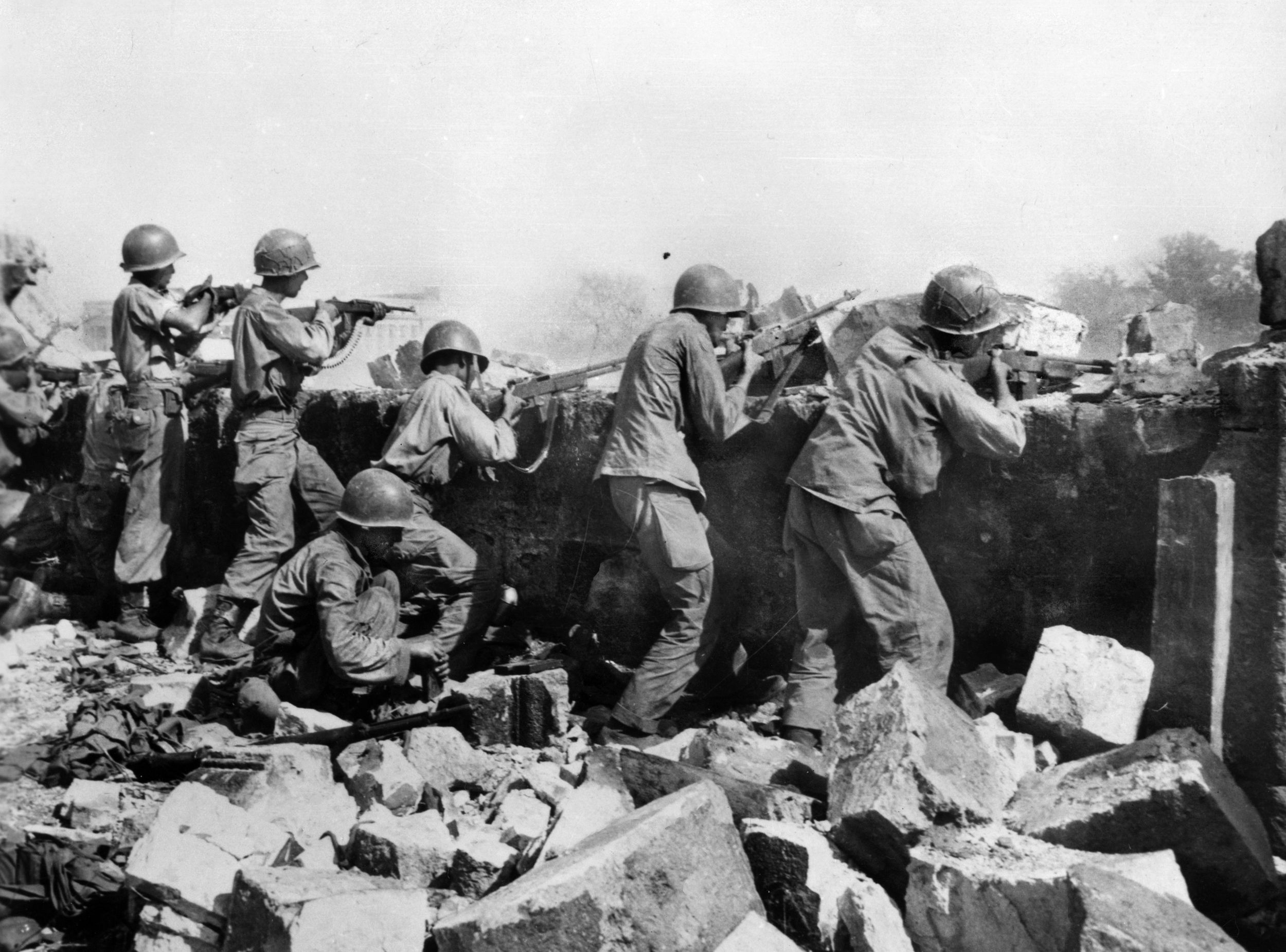This black and white landscape photograph, possibly from World War I or II, captures a stark and desolate warfield scene. It shows six soldiers, each clad in military dress and wearing metal helmets, positioned in the trenches amidst a landscape riddled with large, rectangular chunks of concrete rubble. They are all facing away from the camera, with an assortment of rifles or machine guns, aiming and possibly firing towards an unseen target. A seventh figure is squatting behind them, likely giving orders. The photo's background features a muted grey sky with a subtle tree line, highlighting the somber and meticulous nature of trench warfare. The daylight illumination enhances the gritty realism of the rubble-strewn foreground and the soldiers' tense, focused stances.